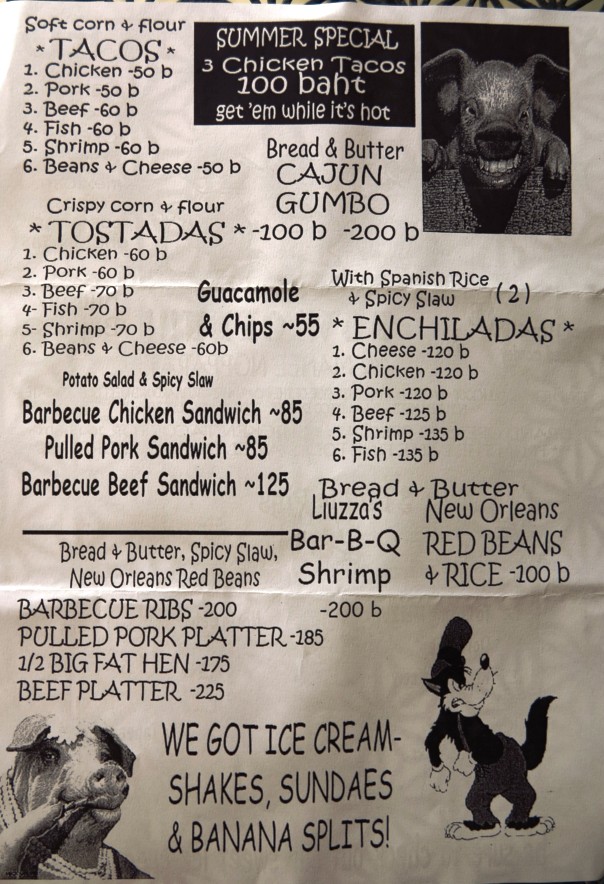Here is the cleaned-up and detailed caption for the image:

---

The image showcases a restaurant flyer, appearing slightly worn with folds and creases on grayish-white paper. At the top, inside a black square, bold text announces a "Summer Special: Three Chicken Tacos for 100 Baht—Get Them While It's Hot." In the upper right corner, there is an unusual illustration of a smiling pig. In the bottom left, another whimsical pig cartoon is seen using a toothpick. The bottom right features a detailed drawing of a cat in a hat alongside a black and white wolf wearing gray suspenders and a top hat.

The menu lists various offerings, including:
- **Soft Corn Flour Tacos:**
   - One Chicken: 50 Baht
   - Two Pork: 50 Baht
   - Three Beef: 60 Baht
   - Four Fish: 60 Baht
   - Five Shrimp: 60 Baht
   - Six Beans and Cheese: 60 Baht

- **Bread and Butter Cajun Gumbo:** 100 to 200 Baht

- **Crispy Corn and Flour Tostadas:**
   - One Chicken: 60 Baht
   - One Pork: 60 Baht
   - One Beef: 70 Baht
   - Four Fish: 70 Baht
   - Five Shrimp: 70 Baht
   - Six Beans and Cheese: 60 Baht

- **Guacamole and Chips:** 55 Baht

- **Enchiladas with Spanish Rice and Spicy Slaw:**
   - One Cheese: 120 Baht
   - Chicken: 120 Baht
   - Pork: 120 Baht
   - Beef: 125 Baht
   - Shrimp: 135 Baht
   - Fish: 235 Baht

- **Potato Salad and Spicy Slaw:**
   - Barbecue Chicken Sandwich: 85 Baht
   - Pulled Pork Sandwich: 85 Baht
   - Barbecue Beef Sandwich: 125 Baht

- **Bread and Butter Spicy Slaw:**
   - New Orleans Red Beans
   - Barbecue Ribs: 200 Baht
   - Pulled Pork Platter: 185 Baht
   - Half Big Fat Hen: 175 Baht
   - Beef Platter: 225 Baht

- **New Orleans Barbecue Shrimp:** 200 Baht
- **Red Beans and Rice:** 100 Baht

At the bottom, in bold capital letters, is a playful proclamation: "WE GOT ICE CREAM, SHAKES, SUNDAES AND BANANA SPLITS."